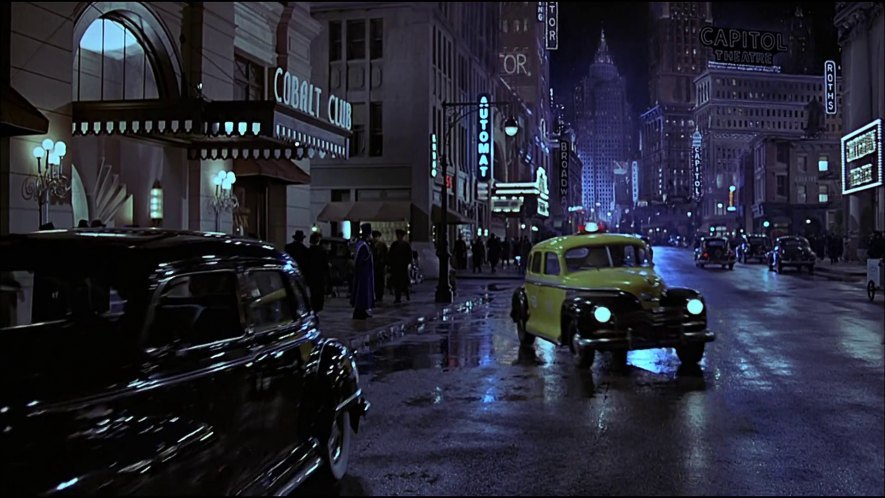The image is a vibrant, color still from what appears to be the 2005 movie "King Kong," set in the 1920s. The scene depicts a bustling night-time cityscape of old New York, highlighted by reflections on rain-slicked streets. Prominently, there are vintage cars, including a swerving yellow and black taxi, alongside a black car. On the left side, pedestrians bustle on the sidewalk next to the Cobalt Club, identified by its black canopy and illuminated archway. In the deep background, there's a tall, pointy-topped building, adding to the vintage metropolis ambiance. Neon signs, such as for the "Automat" and "Capitol Theater," light up the scene, contributing to the overall bluish, cold hue of the image. The street stretches into the distance, lined with tall buildings, providing depth and authenticity to the 1920s setting.